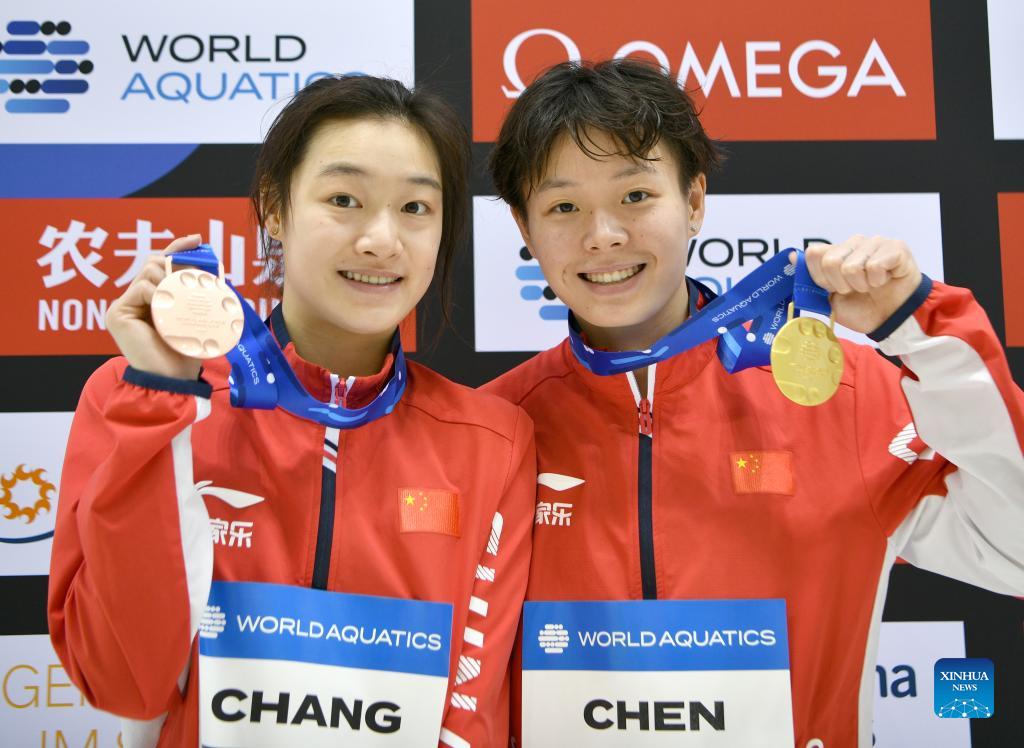The image features two athletes of Asian descent, likely Chinese, standing side by side and proudly displaying their medals. Both individuals are dressed in striking red zip-up jackets adorned with the Chinese flag and a blue banner with white writing that reads "World Aquatics." The woman, named Cheng, is wearing a bronze medal, while the man, named Chen, holds a gold medal. They both have medals strung on blue ribbons and are smiling warmly for the camera. 

Cheng and Chen share similar physical features, including dark black hair and brown eyes, and they appear to be closely related. The backdrop consists of various banners and advertisements, including prominent ones for Omega and World Aquatics, although some of the signage is partially obscured by the athletes. The scene is likely from a prestigious international competition, possibly the World Aquatic Championship, given the context and the medals they are holding.